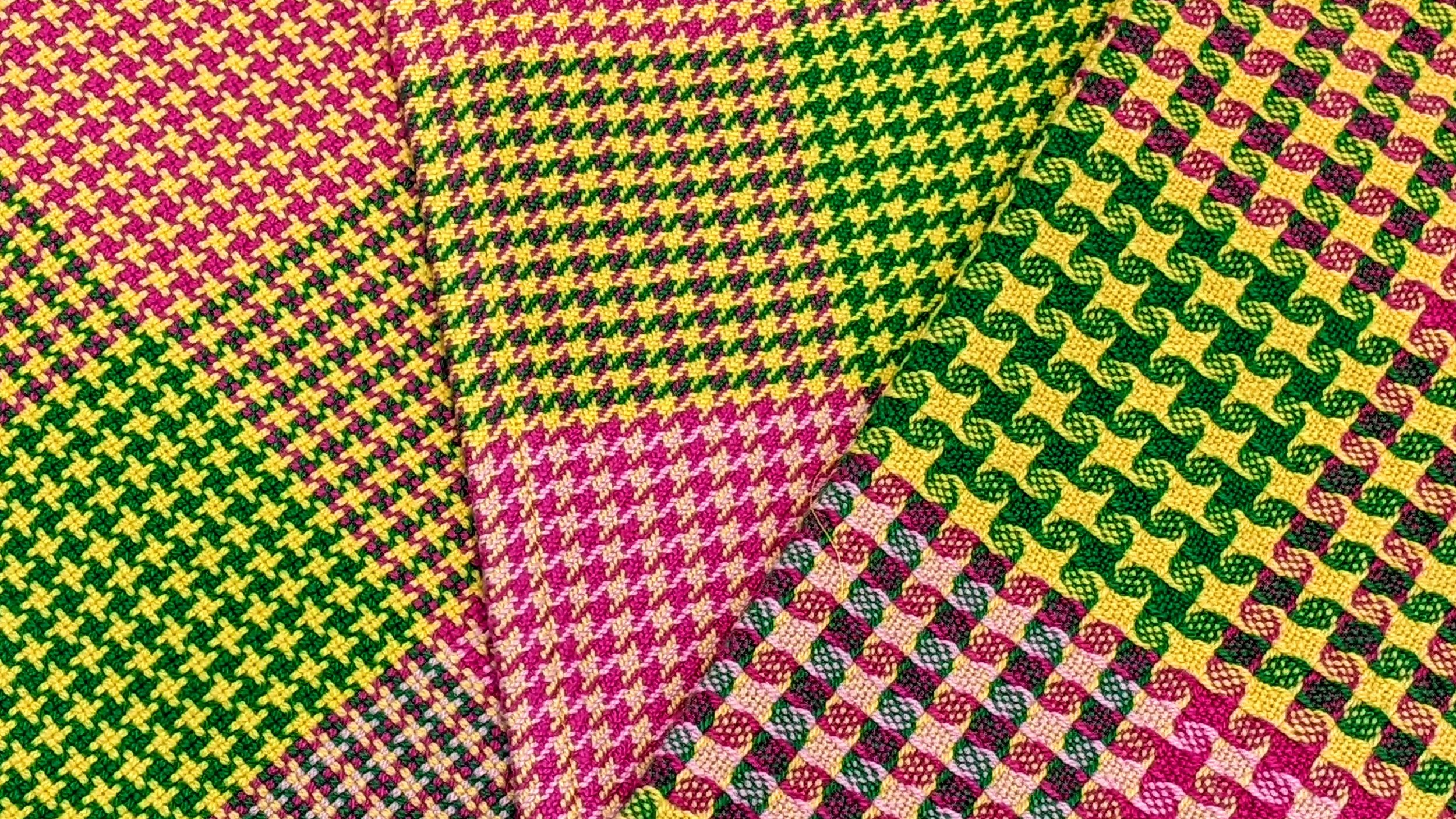The image depicts three vividly colored fabric swatches laid out in overlapping rectangles, each showcasing distinct yet harmoniously colored patterns. Starting on the left, the fabric features a grid of large squares, each containing a smaller cross pattern. The colors include vibrant shades of pink, yellow, green, and purple, with yellow crosses set against varying backgrounds of pink, green, or purple. The middle fabric mirrors the colorful scheme of the left fabric, adorned with large squares each containing a star motif flanked by lines at the top and bottom. The rightmost fabric continues this color palette with intricate rows of small intertwined diamond and spiral shapes, creating a detailed and cohesive visual display. The bright, multi-colored fabrics—possibly designed as tablecloths—bring a cheerful and decorative element to the scene, highlighted by the repeating themes of pink, green, yellow, and purple throughout the patterns. The image captures these textiles in rich detail, emphasizing their complex designs and vibrant hues.